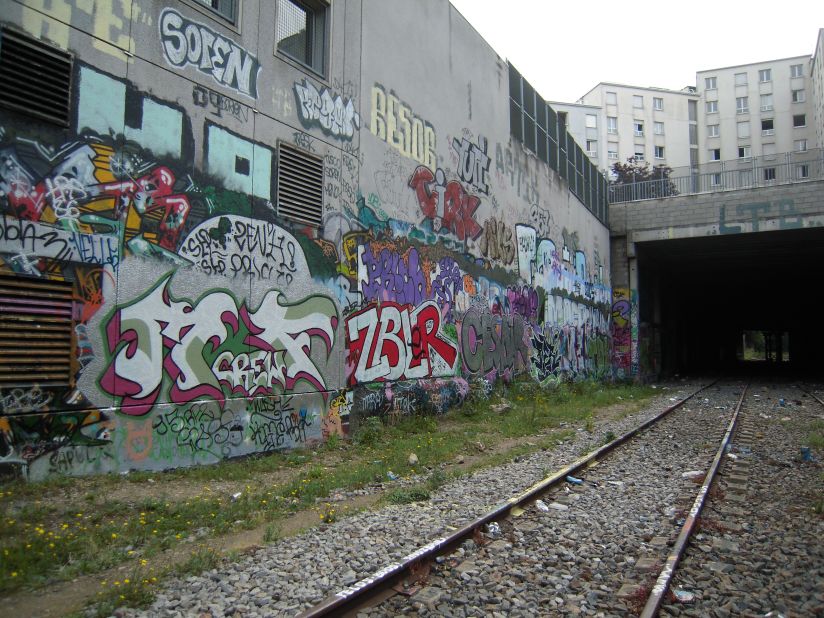In the image, we see an aged, possibly abandoned railway area with train tracks running through a square-shaped tunnel, surrounded by an urban setting. The tracks and the surrounding area show signs of wear, with rust on the tracks and graffiti covering almost every surface. The graffiti features a myriad of colors, including white, green, orange, pink, blue, purple, and yellow, primarily with people’s writings and tags. The grayish concrete walls flanking the tracks are adorned with this vibrant graffiti, creating a stark contrast to the gritty surroundings. Above the tunnel is a gray brick bridge with a silver metal railing, suggesting urban utility. In the background, old multi-story apartment buildings with numerous windows – some of which are open – rise above the scene. The tracks are surrounded by gray gravel, with occasional patches of grass and tiny yellow flowers growing amidst them. A slight scattering of litter is visible on the tracks, augmenting the scene's abandoned feel. Despite the darkness of the tunnel, light filters through an opening at the end, hinting at an unknown destination beyond.